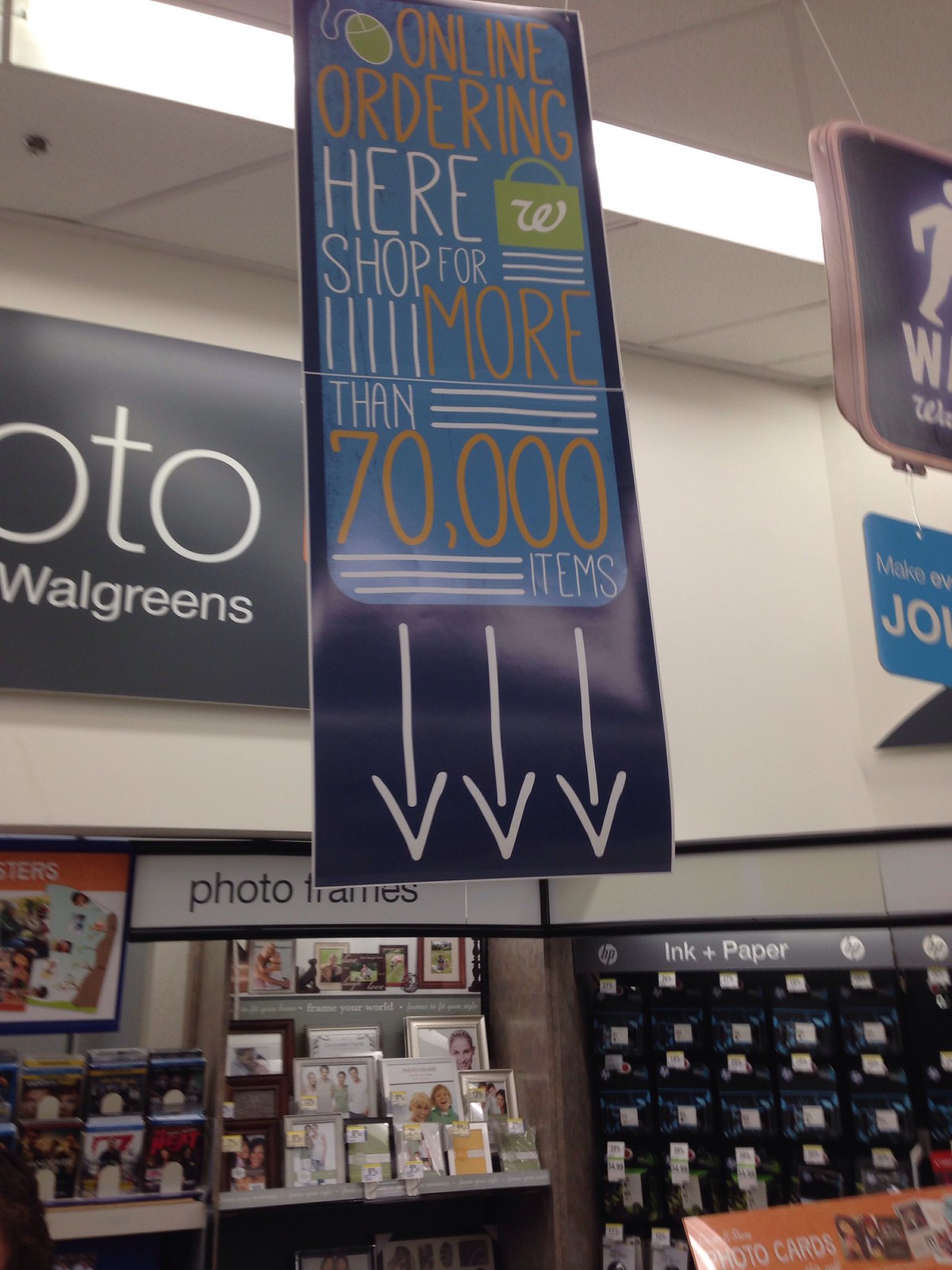This photograph, taken inside a Walgreens store, showcases its photo center. Dominating the foreground is a large blue banner hanging from the ceiling, adorned with playful orange, white, and light green text that reads "Online ordering here, shop for more than 70,000 items." The banner features three white arrows pointing downward and an icon of a green shopping bag with the Walgreens "W" logo.

In the background, a black sign attached to the wall displays the Walgreens name and logo. Below this, shelves neatly arranged with various dimensions of photo frames take up the central part of the image. A white and black sign above these frames clearly labels the section as "Photo Frames." To the left, a collection of DVDs or similar items is visible with distinct cover art. To the right, another shelf holds numerous boxes of printer ink cartridges under a sign reading "Ink + Paper."

The store's drop ceiling, fluorescent lights, and a glimpse of another hanging banner with a stick-figure character complete the scene. This photograph, vertical in orientation, does not include any people, animals, plants, or motorized vehicles.